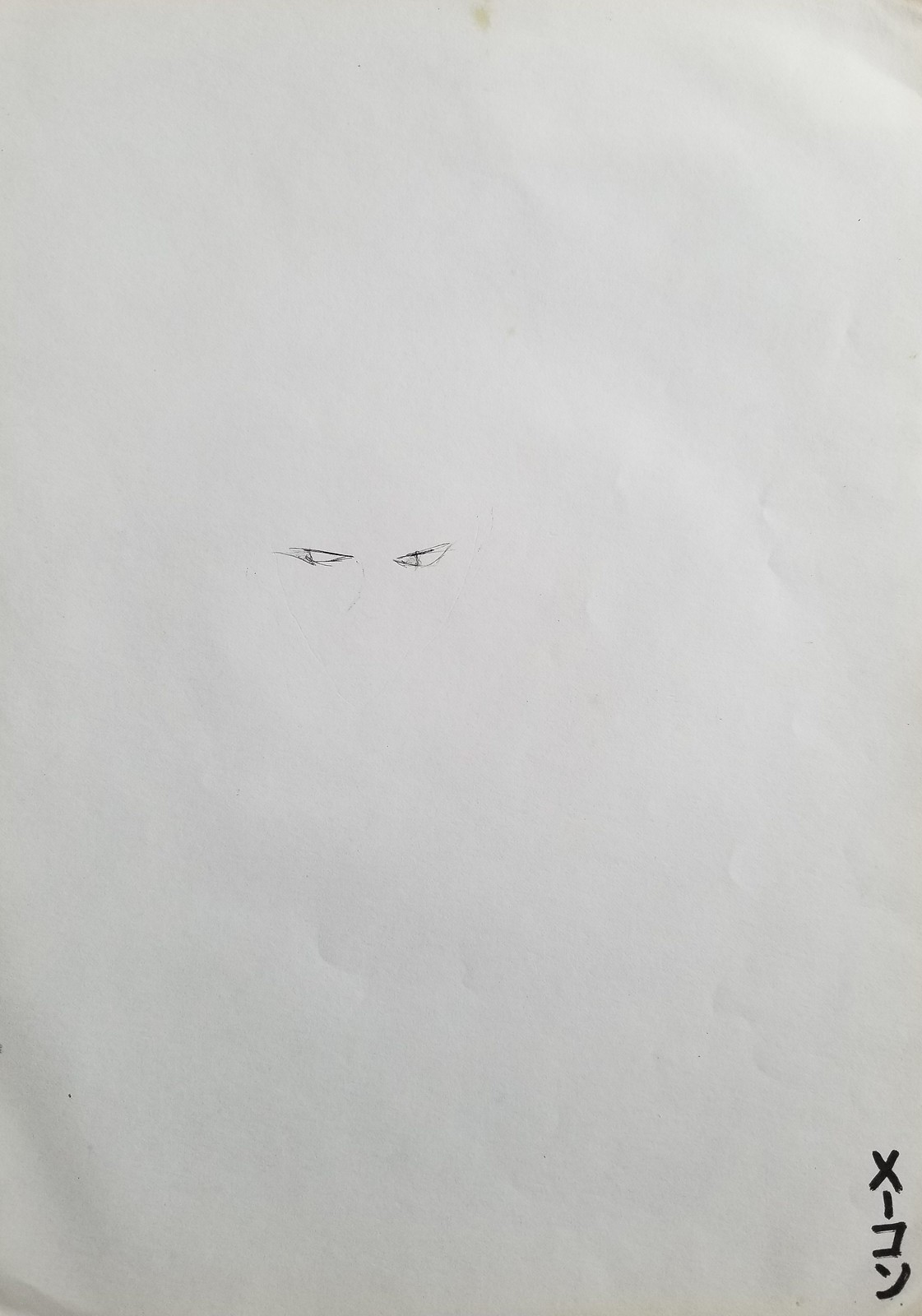This photograph features a worn and slightly creased white piece of paper that appears to have been ripped from a sketchbook. The paper shows signs of wear, including a notable light green stain at the top middle part, and several wrinkles indicative of it having been balled up at some point. At the center of this dingy paper, two narrow and sharply drawn eyes have been penciled in, both irises and pupils subtly directed to the left, giving them a shifty appearance.

In the bottom left-hand corner of the paper, there is a shaded triangular area created with pencil. Meanwhile, the bottom right-hand corner features a series of vertically arranged characters that resemble Japanese or Chinese text. This text consists of a sequence starting with an 'X', followed by a vertical line that appears like a capital 'I', a backwards 'C', and a complex character with a dot and a diagonal line underneath it, ending with what looks like a dot and an angled smiley face. These characters give the appearance of a foreign signature or annotation.